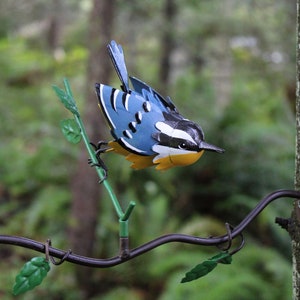The image captures a detailed scene of a plastic bird perched on an artificial branch in sharp focus, set against the soft blur of a forest backdrop. In the background, three vertical tree trunks and numerous green leaves create a serene, natural setting. The foreground features a black twisted rod representing a branch, adorned with green plastic leaves, two of which dangle from the rod. Above, a straight plastic branch with two additional green leaves extends upward, where a blue jay-like plastic bird is situated. This bird, with its black spindly legs gripping the branch, leans out to the right. Its body boasts blue wings with white and black stripes, a blue tail pointing straight up in the center, a yellow stomach, and a distinctive face with white and black streaks. A prominent red chest leads to its thin, pointy black beak, poised as if the bird is ready to take flight into the vivid, leafy backdrop.